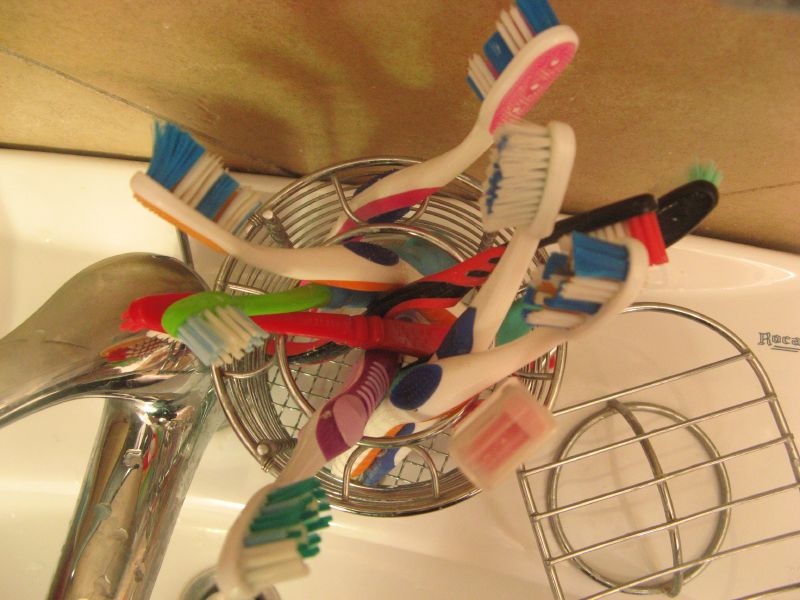This indoor bathroom photo captures a close-up view from above, centered on a wire metal cup filled with a multitude of colorful toothbrushes. Positioned on a white ceramic sink, the cup holds at least eight toothbrushes with varying bristle colors including blue, green, light blue, dark blue, pink, black, orange, and white, one of which has a protective cover. Next to the cup is a silver chrome faucet, which has water droplets on it and a single lever that controls both hot and cold water. Adjacent is a metal grated piece likely intended for a bar of soap. The back wall, appearing tan or light brown like cardboard, sets a neutral backdrop. Part of the sink and the front and sides are partially visible, with the brand logo "ROCA" cut off on the right side. The toothbrushes are reflected in the faucet's shiny surface, adding an extra layer of detail to the photo.